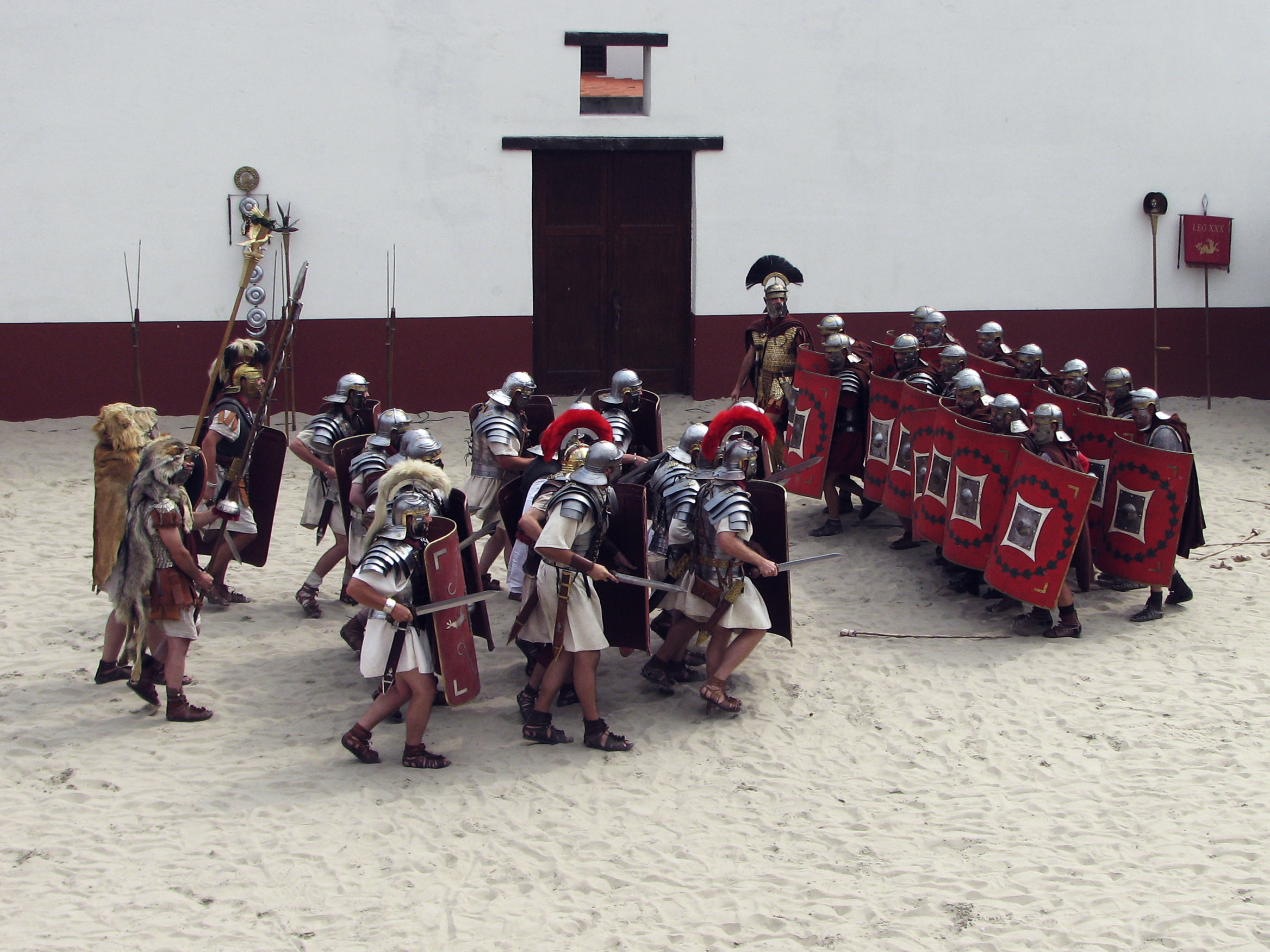The image is a detailed horizontal-rectangular photograph depicting a meticulously arranged replica of a Roman battle scene with figurines on a sandy surface. The setting features a flat, sand-covered area that appears to be part of an arena, characterized by heavily trampled, white sand. In the background stands a tall wall, white with a red lower edge, including a double brown door which adds to the period atmosphere. 

The figures in the scene are predominantly soldiers arrayed in Roman attire, equipped with segmented armor, helmets, and large, curved shields. These shields are red with intricate designs including dark circles forming a large circle, and a white and gray diamond pattern within. To the right, a group of soldiers, their shields covering them from shoulders to shins, seem to be listening to a leader clad in gold metal armor with a distinctive feathered helmet, suggesting a high-ranking officer giving commands.

Approaching this group are additional soldiers, also in Roman uniforms but differentiated by their helmets. They carry swords in one hand and shields similar to their counterparts, indicative of unit cohesiveness. These soldiers sport tunics and sandals, exposing their legs, while behind them, figures in heavier gear with rounded helmets and plate mail can be seen. Collectively, the scene captures the organized clash of two opposing forces, all surrounded by an array of spears, some leaning against the walls, reinforcing the historical reenactment ambiance. In the backdrop, a wooden fence and a dark wood tower with a white roof provide further context, completing the detailed and immersive scene.